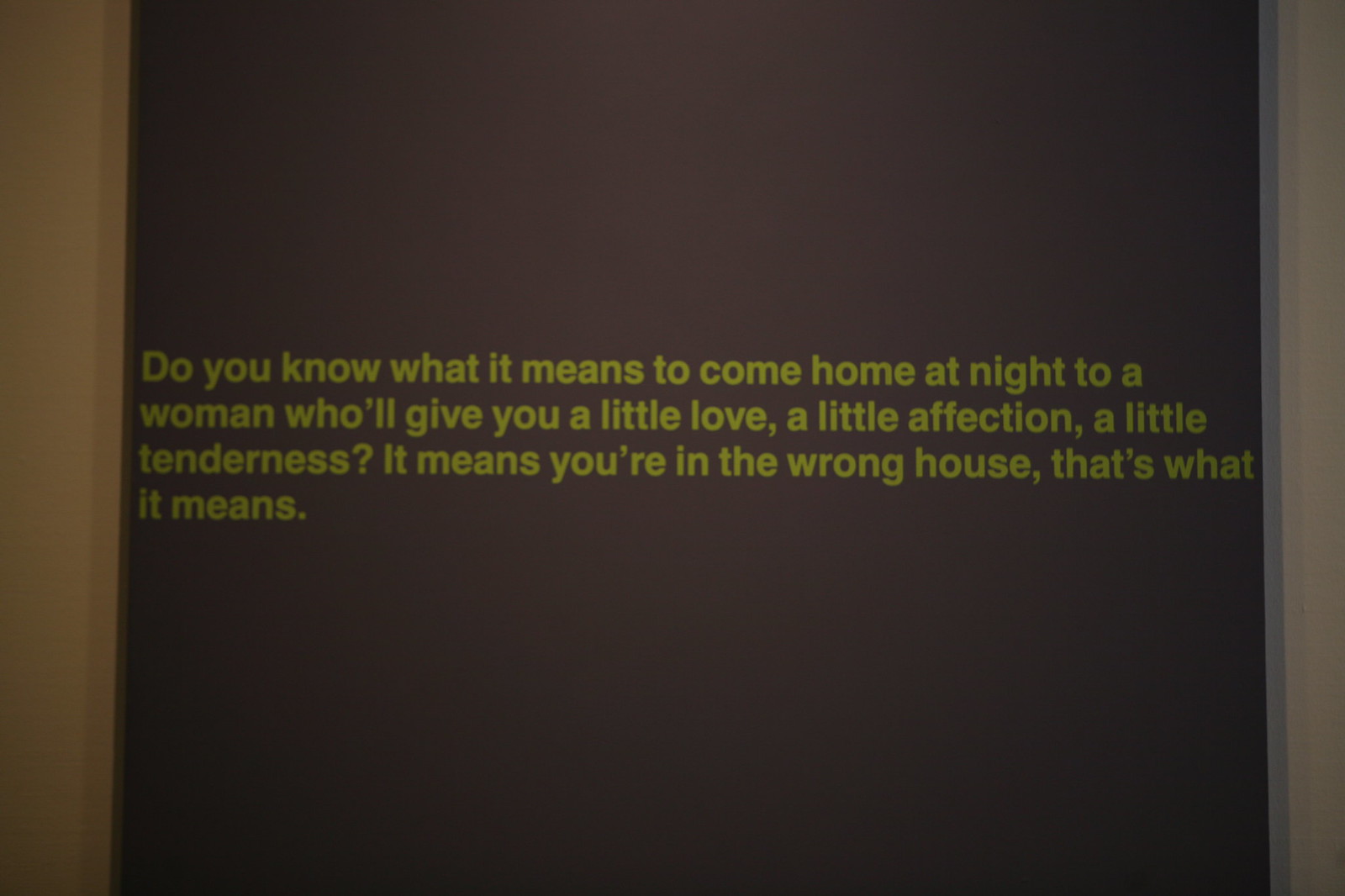The image is a square meme characterized by a predominantly dark brown background with slightly lighter brown vertical bands on both the left and right sides, creating a semi-framing effect. The center of the image, which appears to be a photograph with a bit of realistic blurring, features text in a golden-yellow color that reads: "Do you know what it means to come home at night to a woman who'll give you a little love, a little affection, a little tenderness? It means you're in the wrong house, that's what it means." The overall tone humorously reflects a piece of "boomer humor" suggesting a stereotypical "wife bad" sentiment.